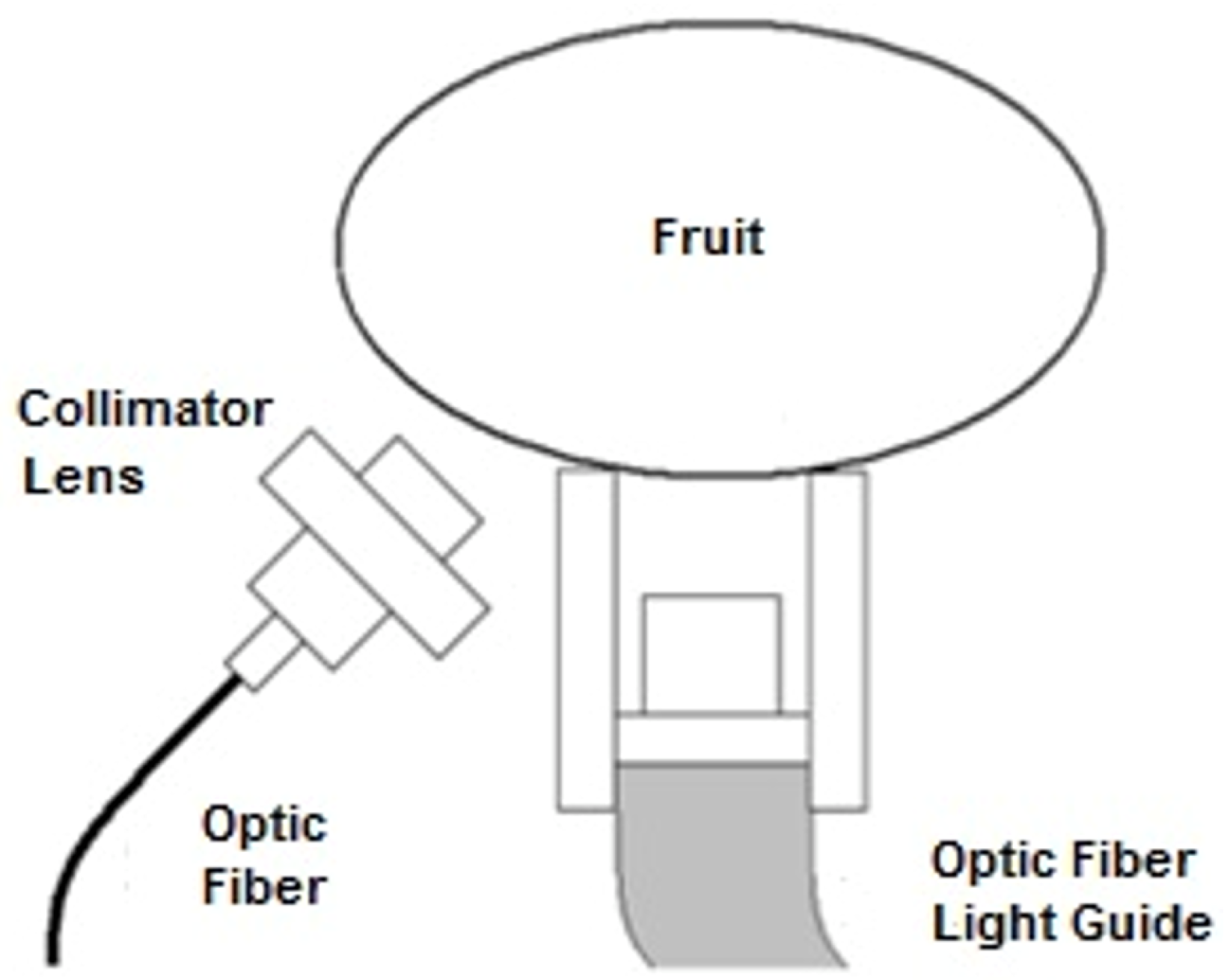In the center of this black and white diagram, an oval labeled "fruit" lies horizontally, with its narrow ends pointing east and west. This oval sits atop two thin parallel pillars with a small square between them, and below the square is a rectangle attached to a dark, filament-like strip extending to the right. Off to the diagram's left, a collimator lens is shown as a series of rectangular shapes arranged in a sandwich-like structure, connected to a long cord labeled "optic fiber." The entire system is identified as an "optic fiber light guide," with this label positioned in the bottom right corner. The background of the diagram is white, emphasizing the stark contrast of the black and gray elements.